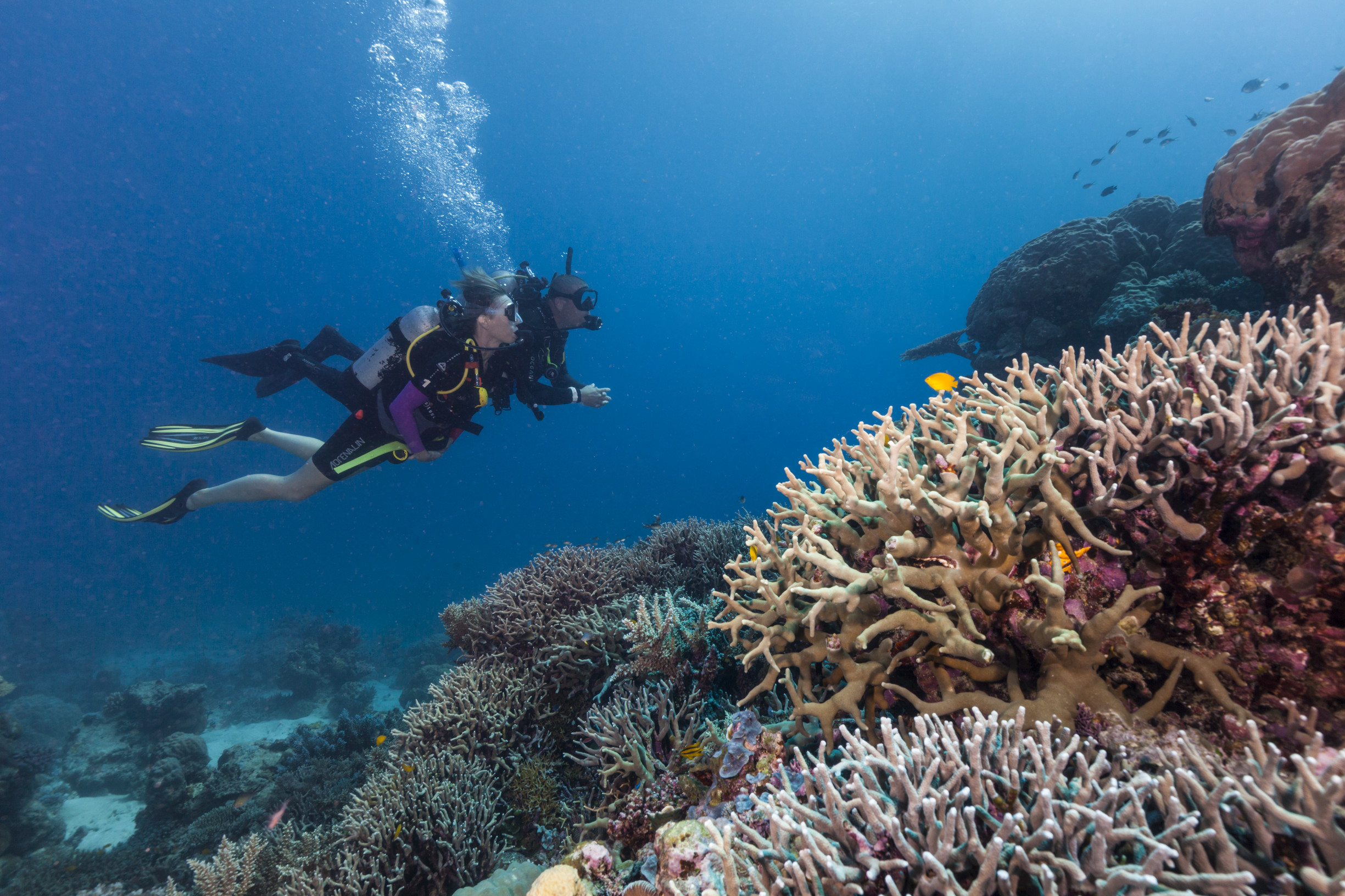In this stunning professional underwater photograph, taken deep beneath the ocean's surface where the water is a dark, rich blue, two scuba divers are captured swimming to the right. The divers, visible from a side view, are enveloped in bubbles from their oxygen tanks. One diver is distinguishable by their yellowish-green flippers and a purple shirt, while the other diver wears all-black flippers. Both are equipped with standard black scuba gear. Surrounding them is a vibrant underwater ecosystem, with a school of fish swimming nearby and a substantial coral reef full of colorful algae—ranging from light purple to tan light brown—spreading out across the ocean floor. Amid the scene, small yellow and orangey fish dart around, adding splashes of bright color to the tranquil, darkening depths. The photograph also features rock-like structures at the top right and intermittent patches of sand scattered along the seabed.